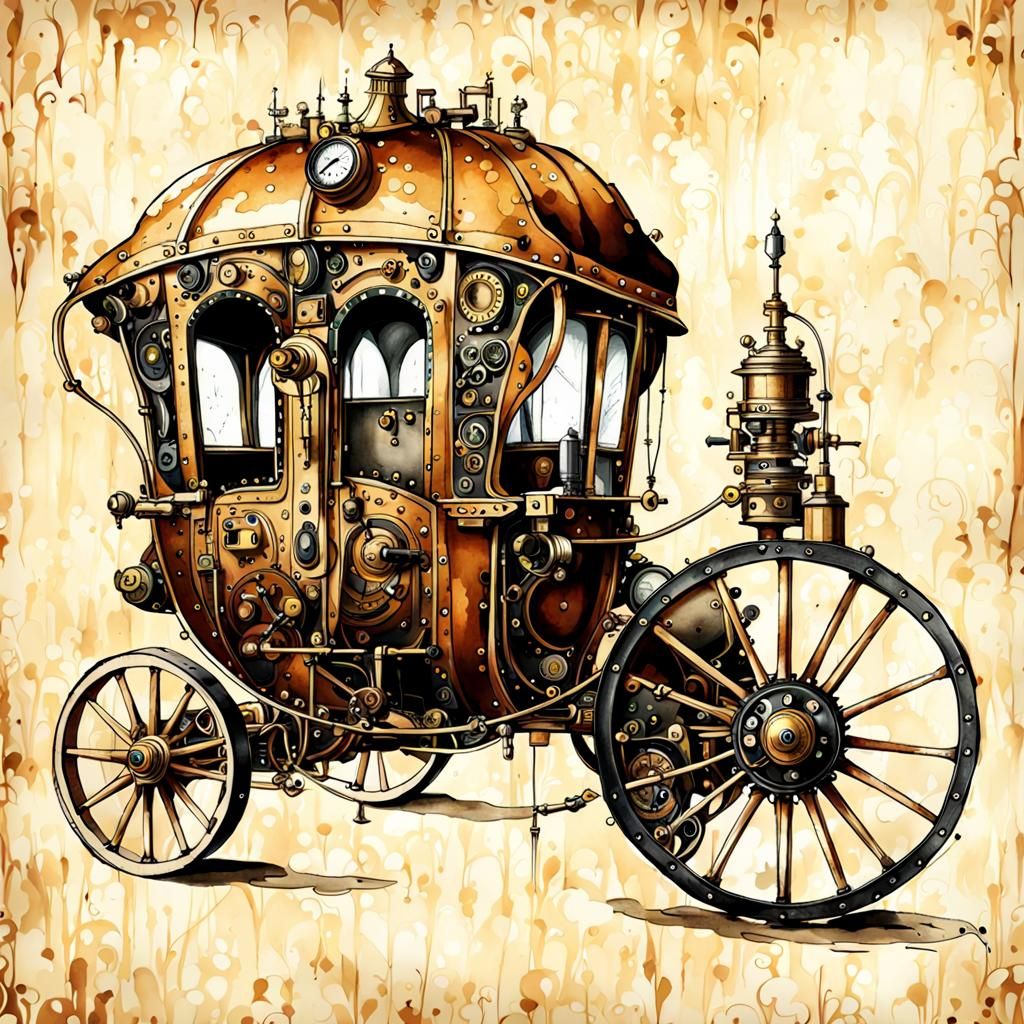In this painting, we see a side-view depiction of a steampunk-inspired, bronze-colored buggy reminiscent of 19th-century Western carriages, but crafted entirely from metal. The buggy features a large front wheel, significantly bigger than the smaller rear wheel, both having distinct black outlines and intricate bronze lines running through them. The wheels are embellished with bolts and screws in black and gold. The front wheel also has a peculiar bolt attached to it, adding to the mechanical aesthetic. The body of the buggy, adorned with various trinkets and gadgets, appears primarily in a coppery-brown hue. Notably, there's a clock or dial situated at the top of the cab with several small objects surrounding it. The background of the painting is textured and abstract, resembling a series of beige and brown brushstrokes or coffee stains, lending an antiquated, worn feel to the piece. The overall scene is rich with detail, blending elements of historical carriage design with industrial, steampunk motifs.